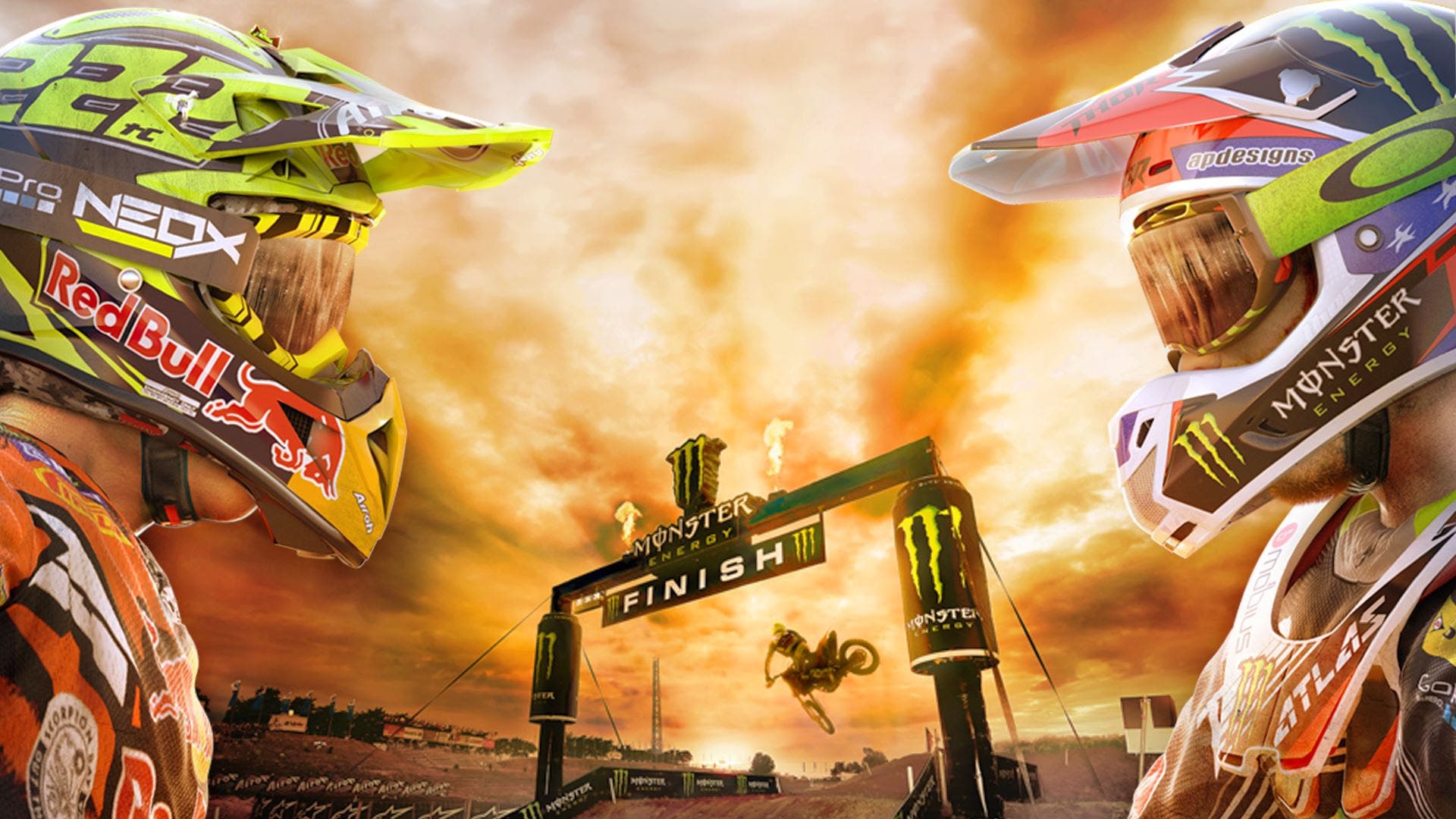The image is a dynamic, computer-enhanced poster for a motocross event, characterized by fiery, cloud-filled skies. Two motocross riders, dressed in full gear with helmets and goggles, are prominently positioned on opposite sides of the image, facing each other. The rider on the left, wearing a yellow helmet branded with Red Bull and Neox, has a Pro-labeled goggle strap. The rider on the right dons a bluish helmet featuring the Monster Energy logo and a chest guard. Centered between them is an exhilarating scene of a motorcyclist airborne mid-stunt, approaching the "Monster Energy Finish" line, marked by large drink cans as poles and a prominent Monster Energy logo overhead. The background vividly depicts a dramatic atmosphere, with clouds appearing ablaze, adding intensity to the event's thrilling ambiance.